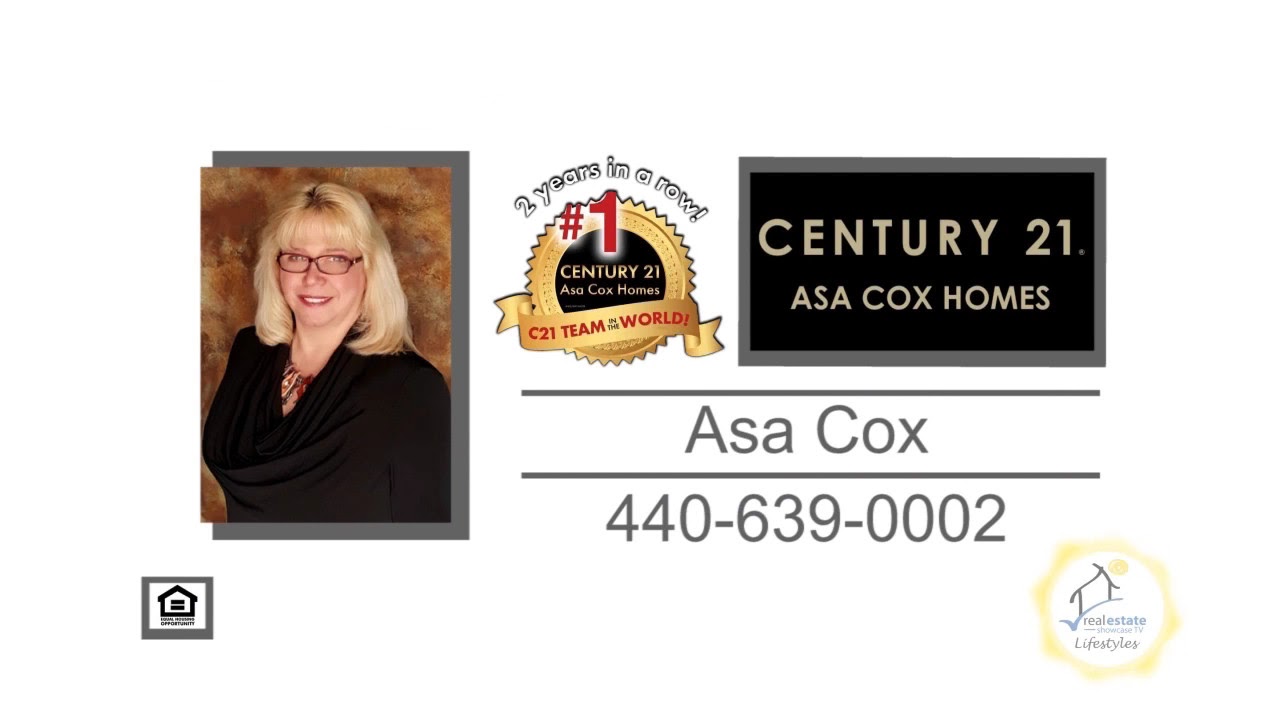The business card predominantly features a white background with various detailed elements. On the left side, there's a photograph of a Caucasian woman with shoulder-length blonde hair, wearing black-rimmed glasses, red lipstick, a black jacket, a brown shirt, and a red necklace. The backdrop for her photo is a mottled brown to beige tone with a gray border. To the right of her photograph, centrally positioned, is a gold seal with a black circular center bearing the Century 21 logo. Around this logo, it states "Two years in a row, number 1." Beneath the logo, the card reads "Century 21 Asa Cox Homes C21 Team World."

Continuing to the right, there's a black box with a gray border that prominently displays "Century 21 Asa Cox Homes." Below this, in gray text, is the name "Asa Cox," followed by the contact number "440-639-0002." Additional details on the card include a gray square with a black cartoon drawing of a house in the far left bottom corner and a gold seal featuring a cartoon house and sun with the words "Real Estate Lifestyles" in the far right bottom corner.